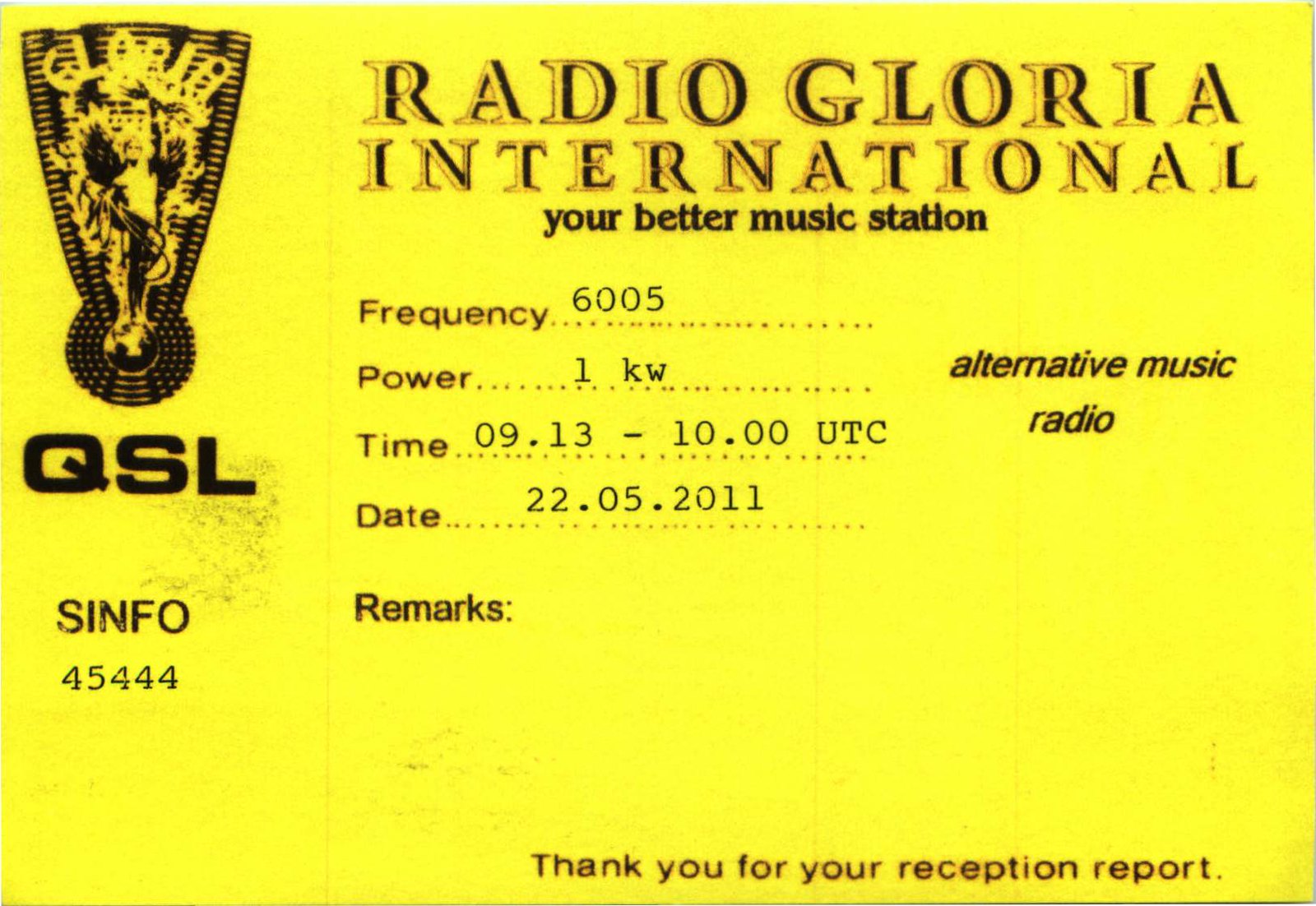The image depicts a bright yellow card with black font, typically sent by radio stations to listeners as a reception report acknowledgment. At the top, it prominently displays "Radio Gloria International, your better music station." The card details the broadcast frequency as 6005 kHz, power as 1 kW, and the broadcast time from 09:13 to 10:00 UTC on the date 22.05.2011. A section labeled "Remarks" is present but left blank. On the right, it mentions "Alternative Music Radio," while on the left, there is a logo with the word "Gloria." Below this logo, "QSL Sinfo 45444" is printed, indicating signal information and reception quality. At the very bottom, the card expresses gratitude with "Thank you for your reception report."